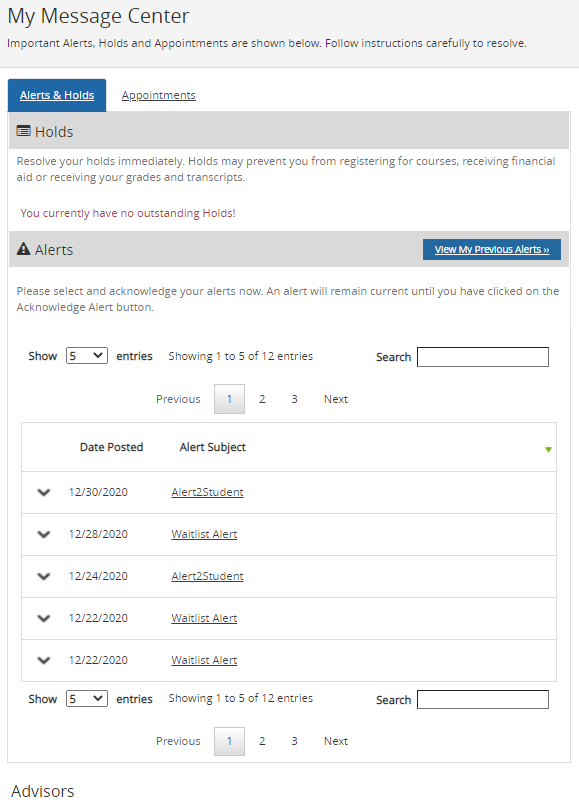The image captures a section of a website, specifically the "My Message Center" page. The title, "My Message Center," is displayed at the top left corner in black text, set against a light gray header background. Below the title, there are two buttons. The first button, labeled "Alerts and Holds," is selected, highlighted by a blue background with white text and an underlining horizontal white line. Adjacent to this is the "Appointments" button, which features black text on a white background, also underlined with a horizontal gray line.

Directly beneath the buttons, a darker gray border spans the width of the section with the word "Holds" written in black text. This section contains detailed information about various holds. To the right of this, another section appears in a middle gray color with the heading "Alerts" in black text. This section lists a series of alerts, sorted by date, beginning with "12-30-2020" and descending to "12-28-2020" and "12-24-2020," among others. 

Below the list of alerts, there’s an option to adjust the number of visible alerts, currently set to show 5 in a white drop-down menu. This selection can likely be changed to different values based on user preference. 

On the right side of the image, there are two white rectangular search bars, allowing for text input or other search functionality.